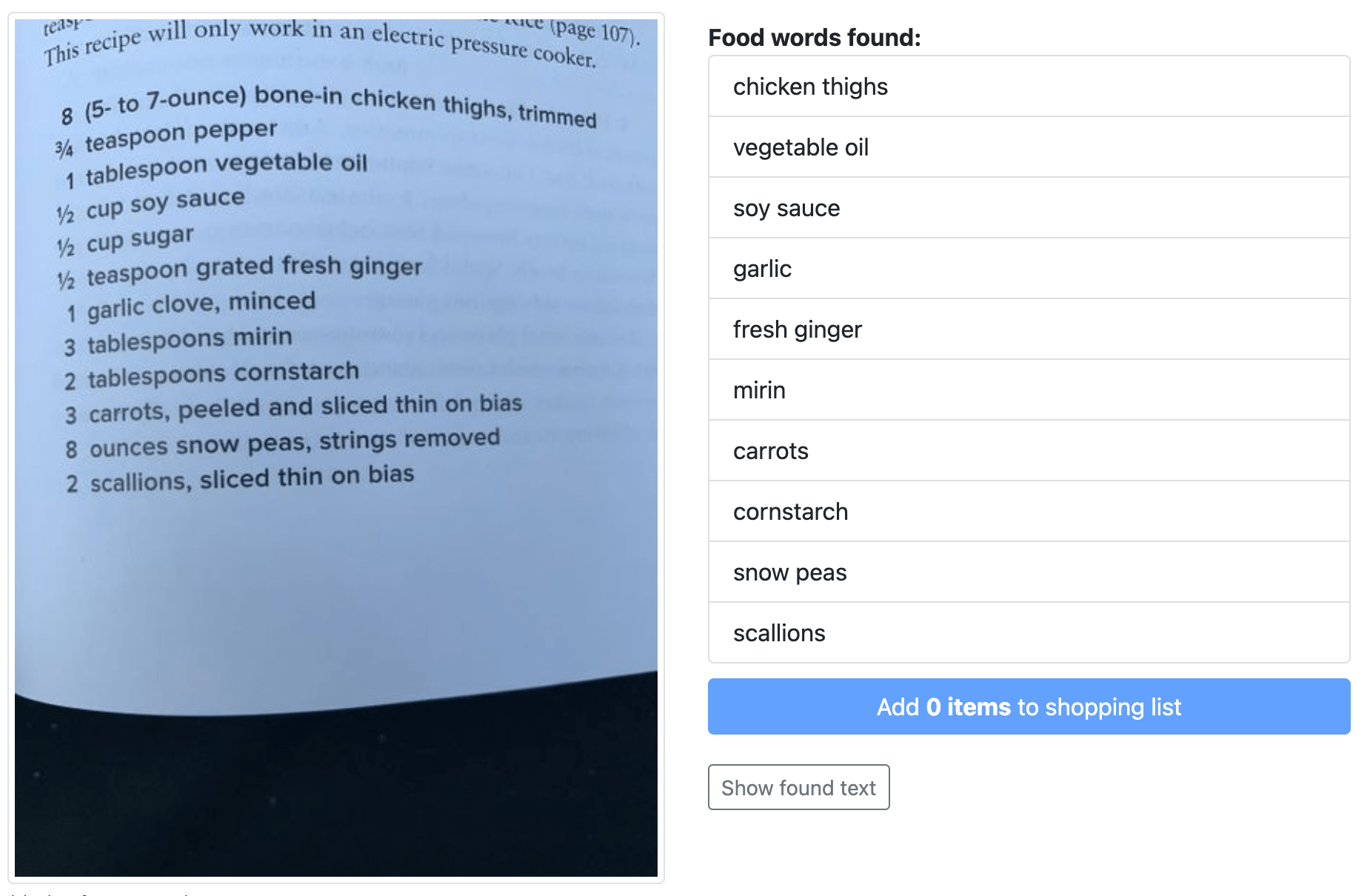The image displays a partial page from a recipe book, with a slight curvature in the page suggesting it might be part of a bound book. On the left-hand side, the recipe is visible under a heading indicating that it is intended for an electric pressure cooker. Above the recipe, the page number "107" can be seen on the right.

The recipe begins with a statement at the top indicating the necessity of an electric pressure cooker. Below this, the title is followed by a list of ingredients in a slightly darker font. Ingredients are listed as follows:

- Eight (5 to 7 ounce) bone-in chicken thighs, trimmed
- Three-quarters teaspoon pepper
- One tablespoon vegetable oil
- One-half cup soy sauce
- One-half cup sugar
- One-half teaspoon grated fresh ginger
- One garlic clove, minced
- Three tablespoons mirin
- Two tablespoons cornstarch
- Three carrots, peeled and sliced thinly on the bias
- Eight ounces snow peas, strings removed
- Two scallions, sliced thinly on the bias

At the bottom of this section is a noticeable white space, with a black background hinting at the end of the page.

On the right-hand side of the image, there is a list under the heading "Food Words Found" in bold, black font. The listed ingredients are each enclosed in a light gray box and include:

- Chicken thighs
- Vegetable oil
- Soy sauce
- Garlic
- Fresh ginger
- Mirin
- Carrots
- Cornstarch
- Snow peas
- Scallions

Below these boxes, there is a blue bar with white text that reads "Add 0 items to shopping list." Adjacent to this, a smaller black box contains the text "Show found text" in white.